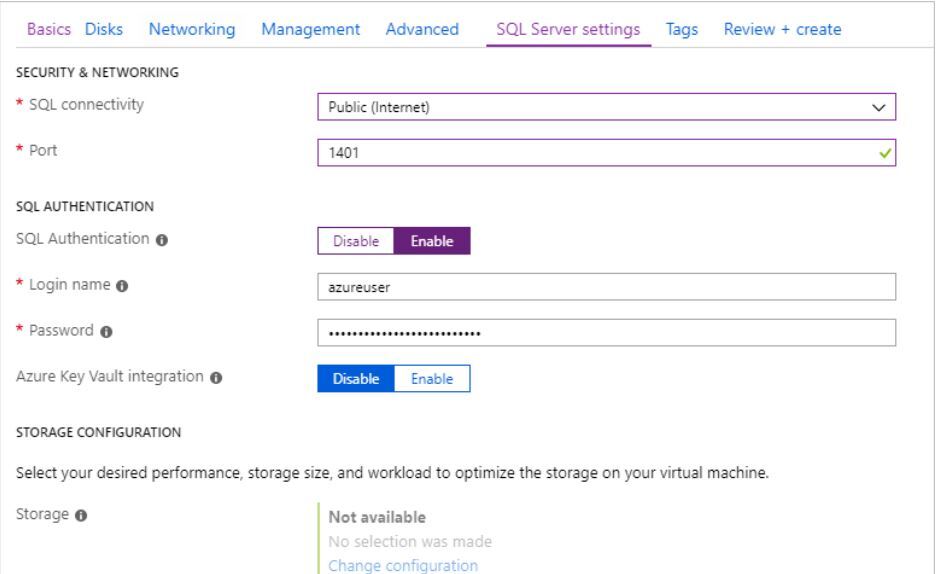The image portrays a computer screen displaying a web-based application or interface. The top section of the interface showcases a series of tabs on a white background, including "Basics," "Disks," "Networking," "Management," "Advanced," "SQL Server Settings," "Tags," and "Review + Create." The "SQL Server Settings" tab is currently selected, indicated by a purple underline, while the "Basics" tab is highlighted in purple.

On the left sidebar, the options "Security" and "Networking" are listed, with sub-options for "SQL Connectivity and Port" and "SQL Authentication" displayed in darker font. This section includes an information icon next to "SQL Authentication," and fields for "Login Name" and "Password." Additionally, there are options for "Azure Key Vault Integration" and "Storage Configuration."

In the main settings area, various choices are indicated: "Public" internet visibility is selected, the port number "1401" is specified, and a feature has been enabled with the username "azure user." A subsequent selection to disable a feature indicates an action being taken by the user.